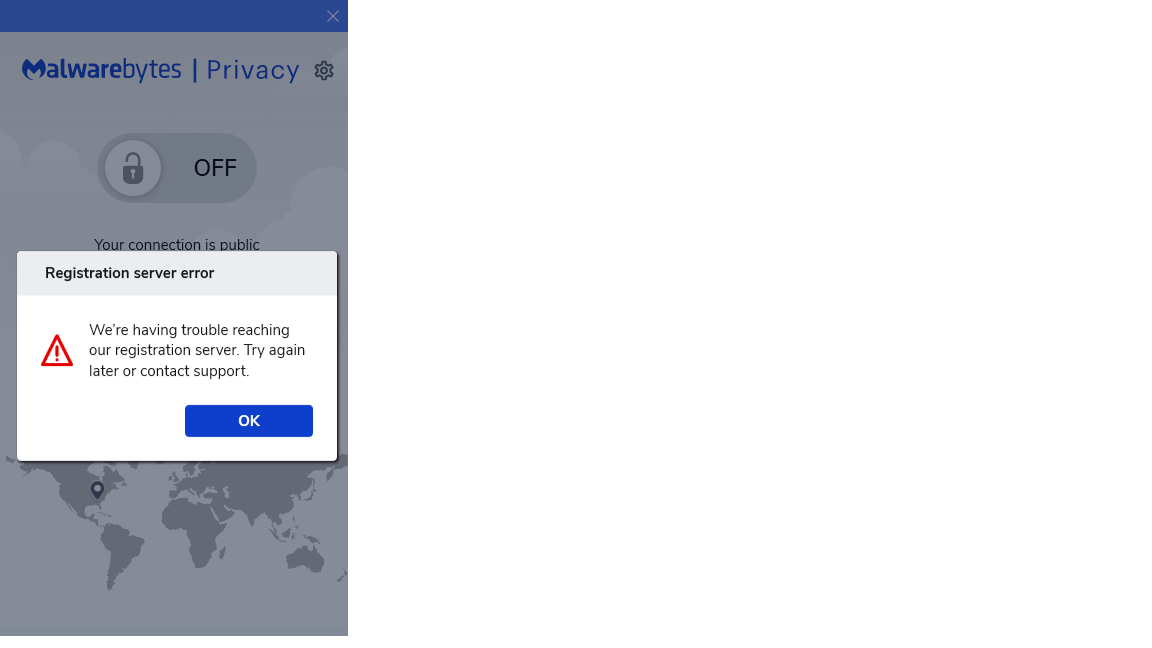The image shows a screen interface with multiple elements. At the very top, a blue bar runs across the width of the screen. In the top-left corner of this blue bar, there's an 'X' sign. Below the blue bar, the rest of the background transitions into a mixture of grey and white hues.

Directly beneath the blue bar, the title "Malwarebytes" is prominently displayed in blue text. A thin line separator follows the title. Next to the title, the word "Privacy" can be seen, also in blue, accompanied by a settings symbol.

Centrally located on the screen is a large, curved grey cylinder. On the left side of this cylinder is a white circle that contains an unlocked grey lock symbol. On the right side of the cylinder, the word "OFF" is written in black, uppercase letters. Below this cylinder, in dark grey text, there is a message that reads "Your connection is public."

A small warning pop-up box is present on the screen. At the top of this box, within a light grey bar, is the message "Registration Server Error" in black text. The rest of the pop-up box has a white background. To the left, there's a red triangle with an exclamation point inside, signaling an error. The message reads, "We're having trouble reaching our registration server. Try again later, or contact support," in dark grey text. In the bottom-right corner of the pop-up box, there's a blue rectangle with curved corners, containing the word "OK" in white, uppercase letters.

Below the pop-up box, a picture of a map is partially visible, showing a location symbol pointed towards Florida.